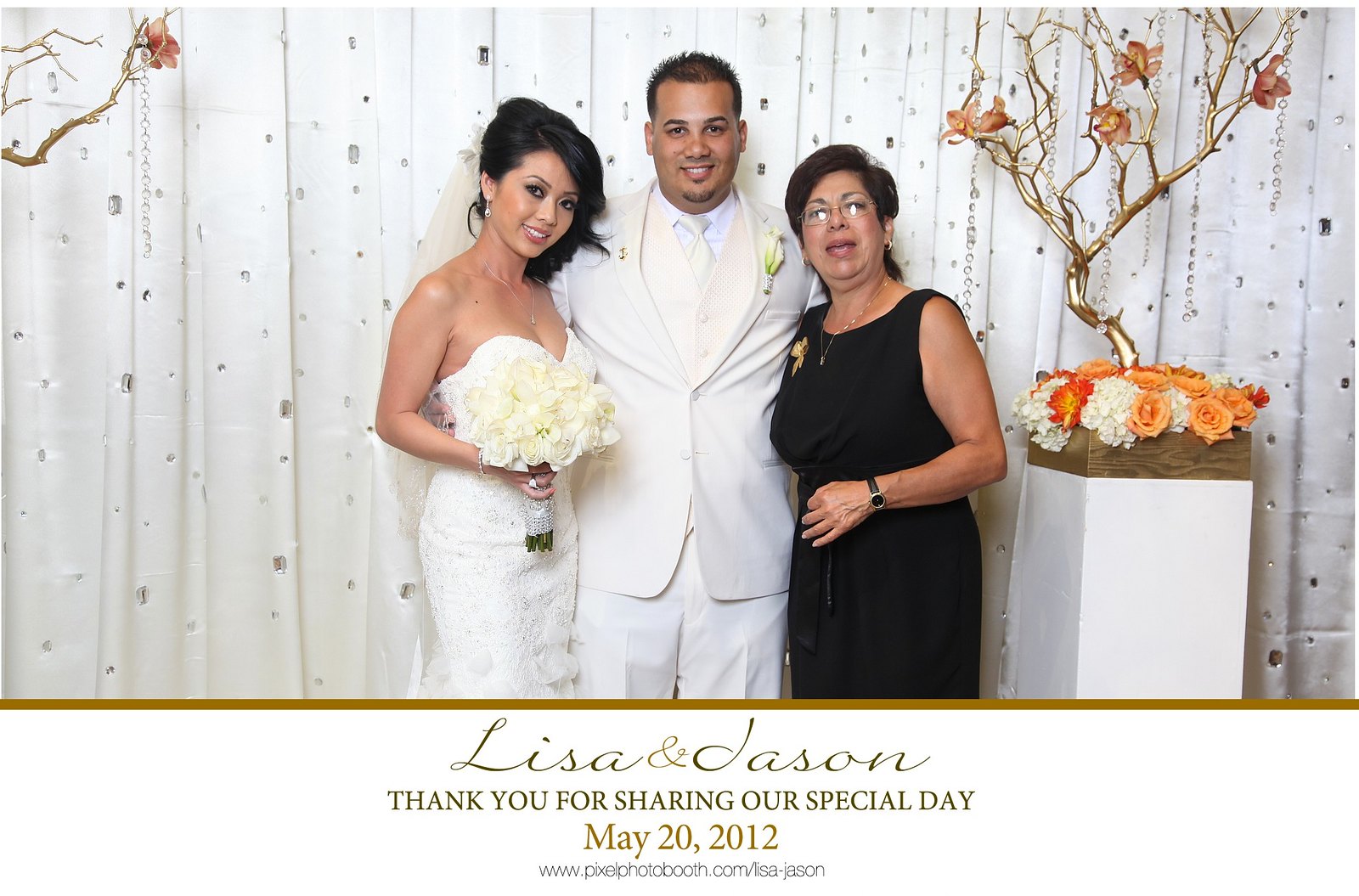This horizontally aligned rectangular photograph captures an intimate wedding moment featuring a bride, groom, and their mother against an elegant backdrop. The bride, positioned on the left, wears a sleeveless white lace gown and holds a bouquet of white flowers in her right hand. Her left arm lovingly encircles the groom. She has long black hair and is smiling radiantly. The groom, standing in the middle, sports an all-white suit with a white tie and short black hair. He shares a joyful smile, indicative of his happiness. To his right stands the mother, dressed in a sleeveless black dress and wearing glasses. She has her hair pulled back and complements her attire with a black wristwatch. Her right arm is affectionately around the groom. The background features a white curtain embellished with silver decor and possibly rhinestones. In the upper left corner of the image, a golden tree branch adorned with flowers and beads can be seen. To the right of the mother, a white table is set up with orange and white flowers on top, accentuated by another gold tree branch. The bottom of the picture is bordered with a thick gold frame, which bears the inscription: "Lisa and Jason, thank you for sharing our special day, May 20th, 2012."